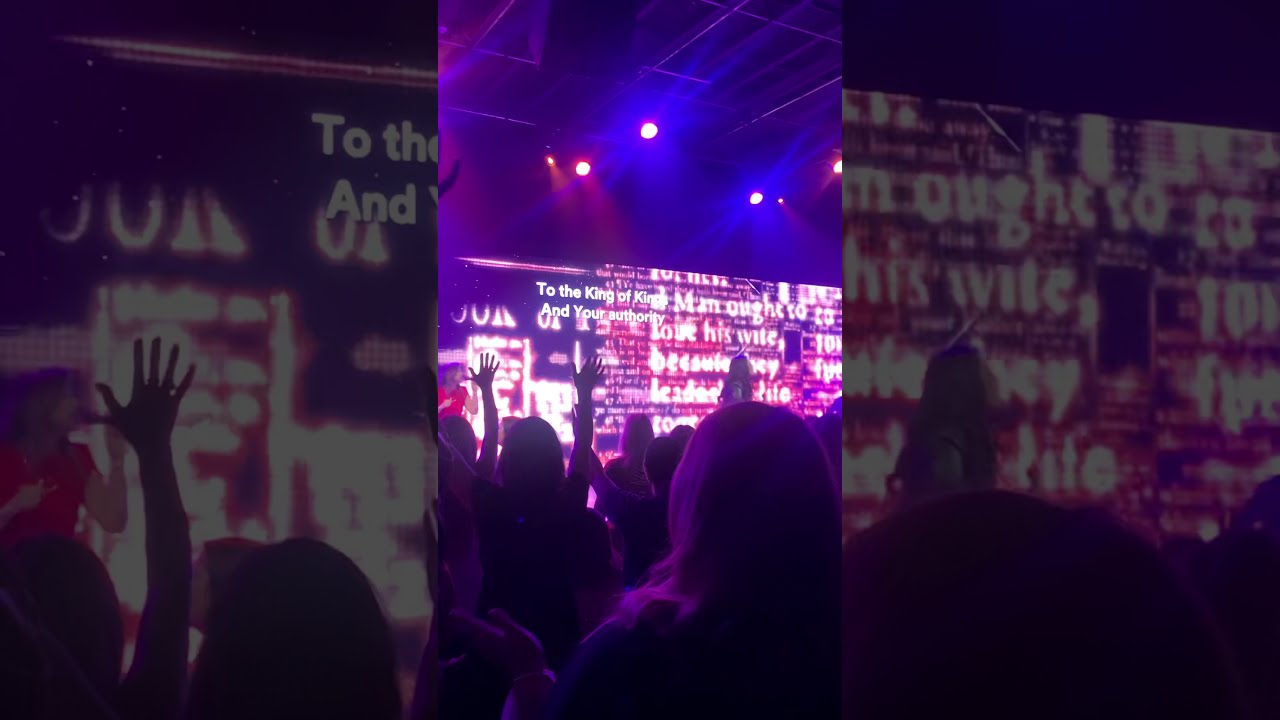The image depicts a Christian concert or worship event, captured in a central vertical rectangular bar, flanked by background segments showcasing the same scene at varied zoom levels, with a dark filter applied. The crowd, predominantly women, has their hands raised in worship, bathed in a mix of purple, blue, and red light from overhead spotlights. A female singer, dressed in a red shirt, accompanied by guitarists, performs on stage in front of a large LED screen displaying song lyrics. The atmosphere is vibrant, echoing the communal spirit of the event.